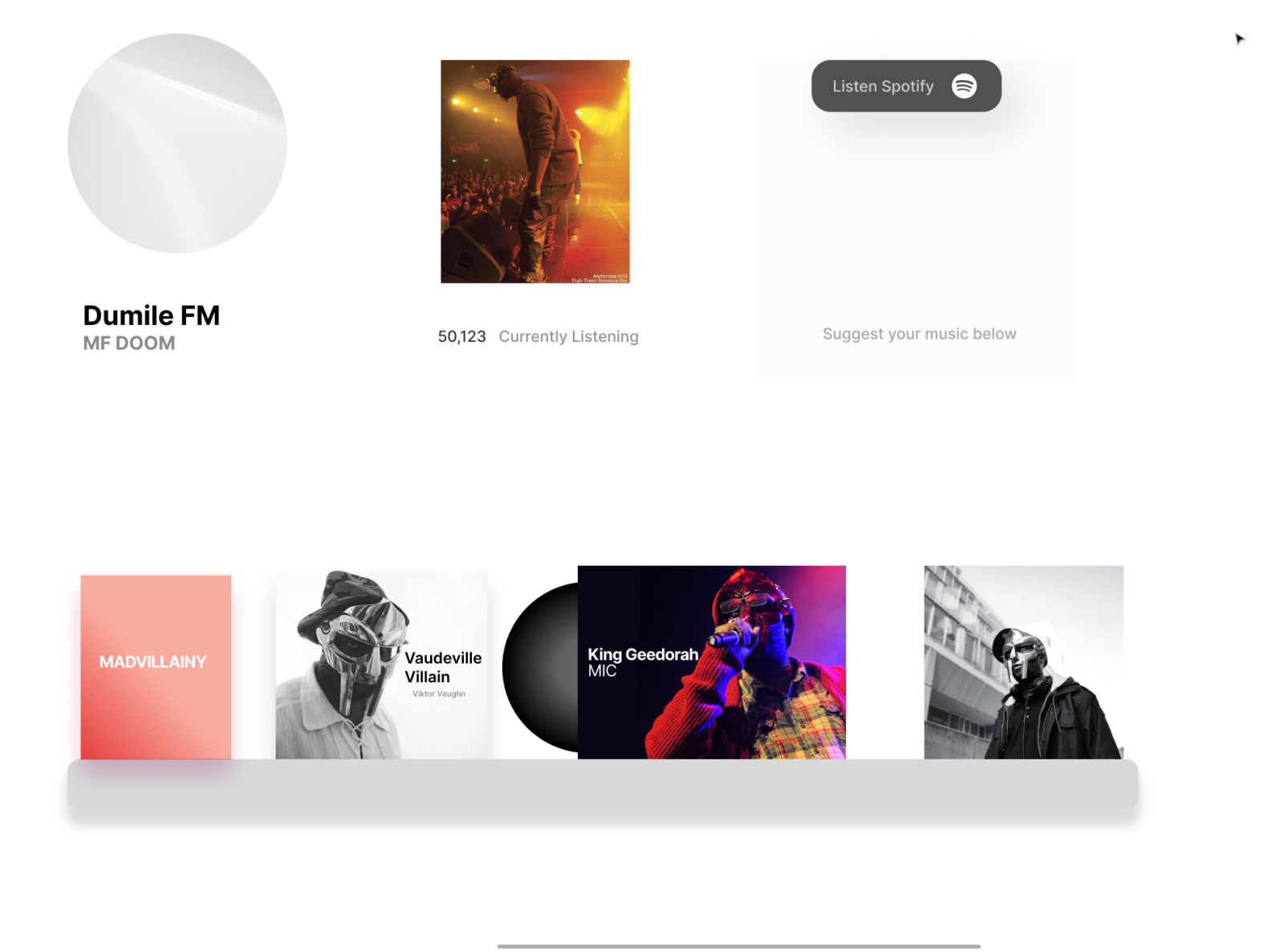This image is a screenshot of a website featuring a clean, white background. The layout is organized into two rows, each containing three distinct panels. 

**Top Row:**
1. The first panel displays a circular image in various shades of gray. Below the circle, the text "DUMILFM" is prominently featured in uppercase letters.
2. The second panel captures a singer on stage, looking down at the audience. This section includes the text "50,123 currently listening."
3. The third panel showcases another singer at the top and contains a call-to-action button that reads "Listen on Spotify." Below this button, the text instructs users to "suggest your music below," and lists three music titles: "Mad Villainy," "Vaudeville Villain," and "King Jidora M.I.C."

**Bottom Row:**
1. The first panel features a graphic of a man walking down a street wearing a mask.

At the bottom of the image, there is a light gray border followed by a white space with a thin line separating it from the rest of the content.